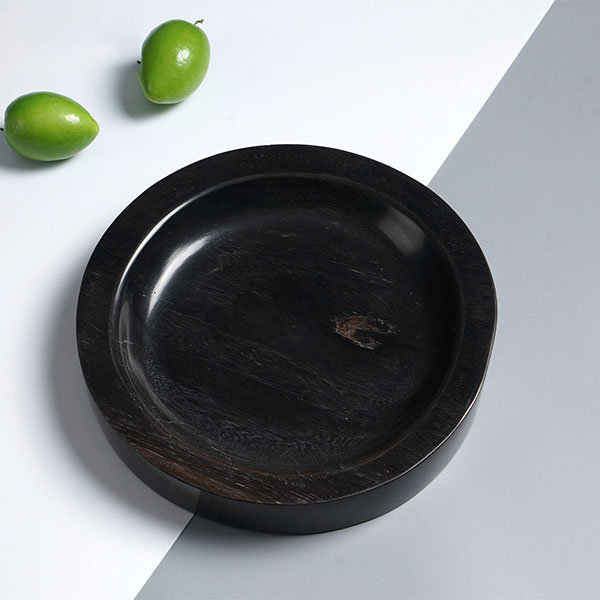The image features a shallow black bowl, reminiscent of an ashtray but lacking the typical sections for holding cigarettes, sitting on a table that is diagonally divided into white and light gray or lilac parts. The bowl appears to be made of wood, stained a glossy black, displaying some worn black-brown spots and visible wood grain. Above the bowl, situated on the white section of the table, are two green oval-shaped fruits, possibly olives or unripe walnuts still in their hard, cream-colored casings. The stark photograph captures the interplay of light and shadow on the worn, glossy surface of the wooden bowl and the vivid green of the fruits.